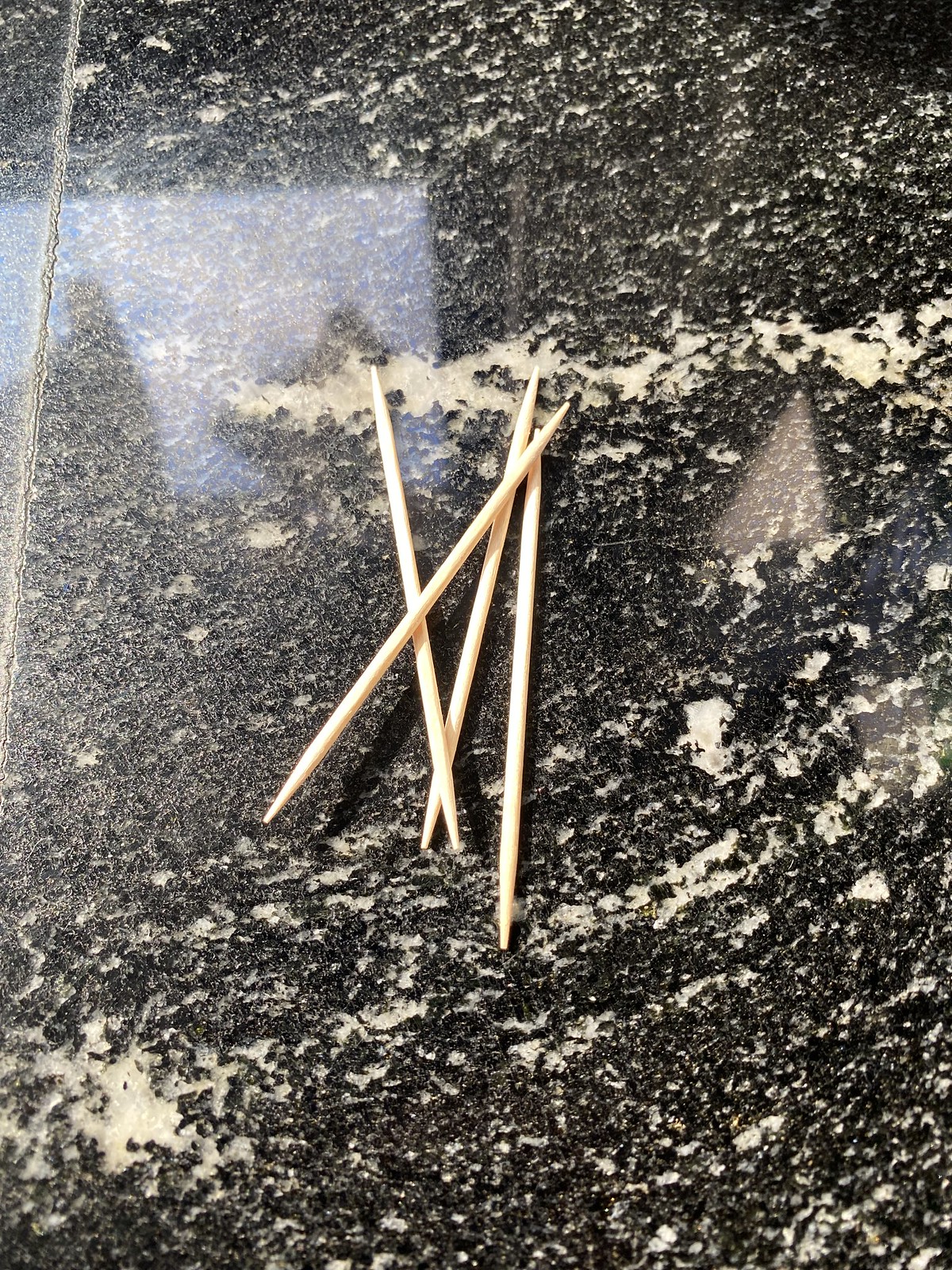The image depicts a close-up view of smooth, glossy black and white marble, resembling a kitchen countertop. Atop this sleek surface, a cluster of beige bamboo skewers is arranged in a seemingly haphazard manner. The skewers overlap each other, creating intricate intersections: the two at the bottom form an 'X'; another skewer stands upright beneath the main diagonal skewer running from the right to the left. The uppermost skewer lies horizontally across all others, adding to the dynamic crisscross pattern. This detailed arrangement combines to form a visually interesting composition against the polished marble backdrop.